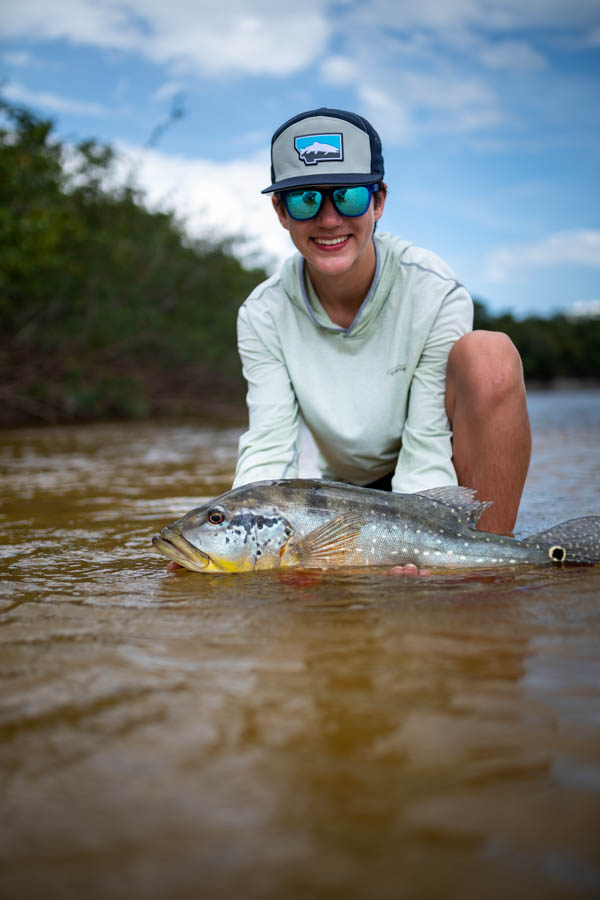The image captures a close-up scene at a river's edge, depicting a young person waist-deep in muddy water. The individual, wearing reflective blue sunglasses and a white, long-sleeved sun shirt, is crouched down with one knee bent and visible, positioned to the right of the frame. They are holding a large silver bass fish with thick, yellow-accented features just above the water's surface. Adorned with a dark blue or purplish baseball cap, featuring a white center with the outline of a state and a mountain image on it, the young person is smiling, revealing their top teeth highlighted by red lips. In the backdrop, a vivid blue sky filled with scattered white clouds stretches above a line of large, dark green trees that run along the riverbank, enhancing the outdoor and adventurous atmosphere.